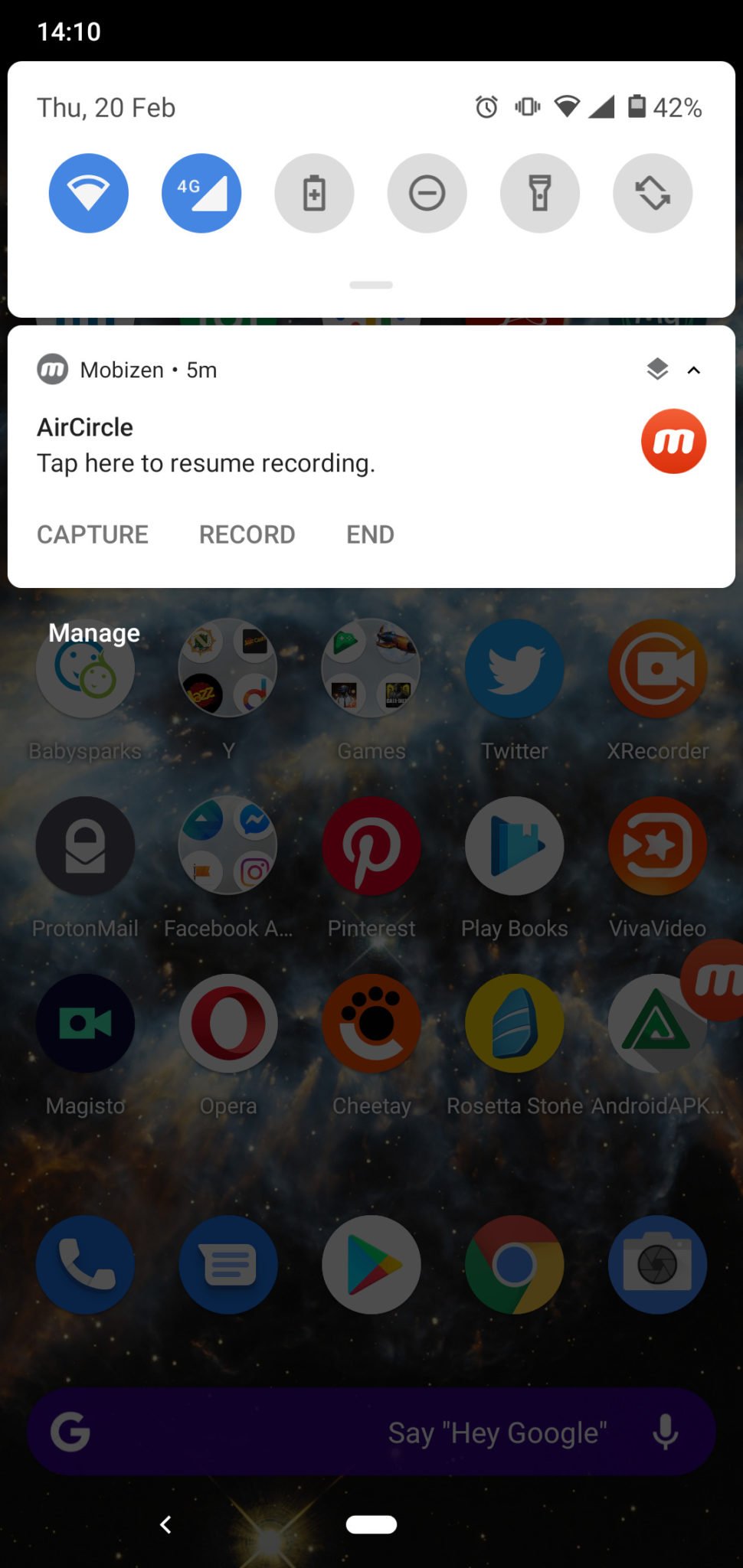In this cell phone screenshot, the top of the image displays a black border with white text indicating the time as 14:10. Below, it reads "Thursday, February 20th," alongside various status icons, including the date symbol, Wi-Fi signal strength, and battery level at 42%. Further symbols include a circle with a fan-like shape, a blue circle, a trash can icon, a battery symbol, and additional icons. There is text reading "must have been five minutes, air circle type, here to resume recording, capture, record, end." The main portion of the image shows the home screen of a cell phone, slightly dimmed. Various installed apps are visible, including Pinterest, Twitter, Facebook, Play Books, VivaVideo, Majestic, Opera, Cheetah, Rosetta Stone, and Chrome. The screen also features the "Say Hi to Google" prompt.